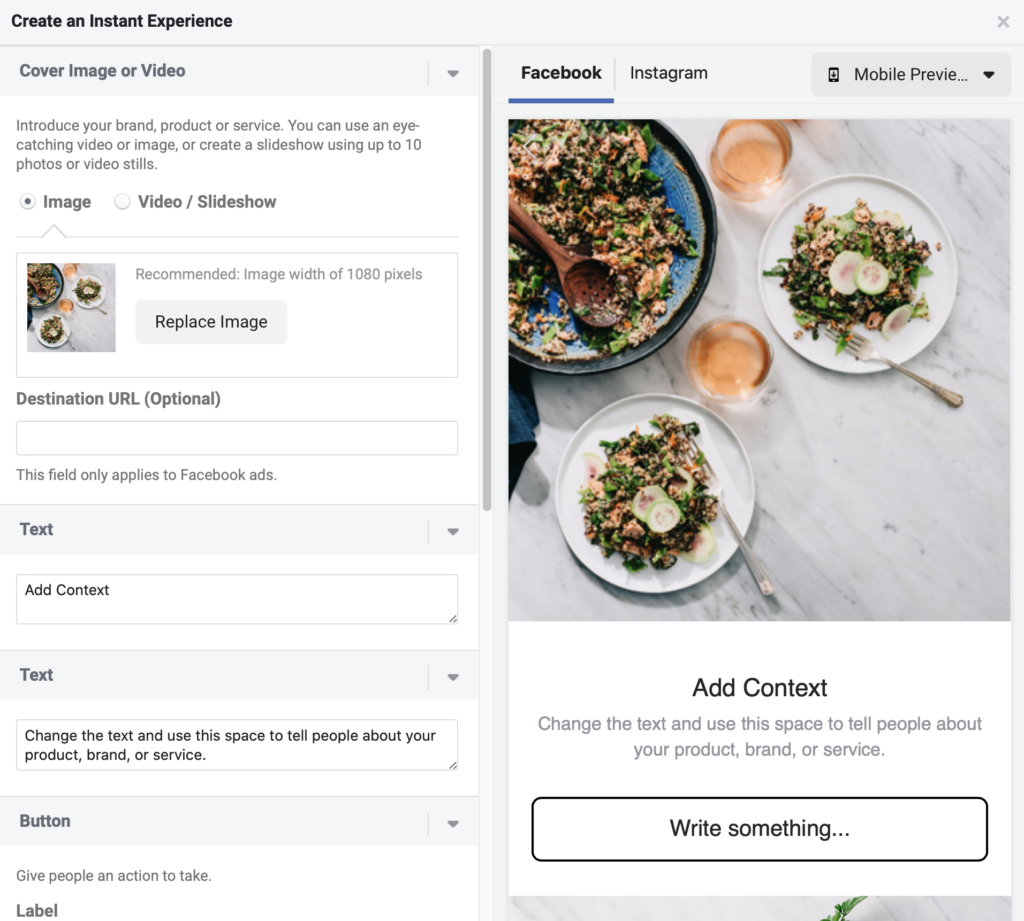The image displays an interface for creating an instant experience, split into two main sections. At the top left, a heading reads "Create an Instant Experience." Below this, there is an option for a cover image or video, with "Image" currently selected. Underneath this selection, an image is shown featuring simple dishes and plates of food, including what appears to be meat and vegetables. 

To the right of the image, there are radio buttons offering a choice between "Image" and "Video/Slideshow." Below the image upload section, there is a box labeled “Destination URL,” which is currently left blank and marked as optional. 

Next, there are sections for adding text. One box displays placeholder text saying "Add Context," indicating no text has been added yet. Another text box prompts the user to "Change the text and use this space to tell people about your product, brand, or service," suggesting this space is intended for a longer text description.

A button option allows users to add a button or label. On the right side of the interface, there's a preview area showing how the content will appear on Facebook and Instagram, currently displaying a mobile preview on Facebook. Below the preview, there's another section to add context or write something.

The overall interface is designed to be user-friendly, allowing the creation of engaging content using images, videos, and descriptive text with a live preview feature for social media platforms.